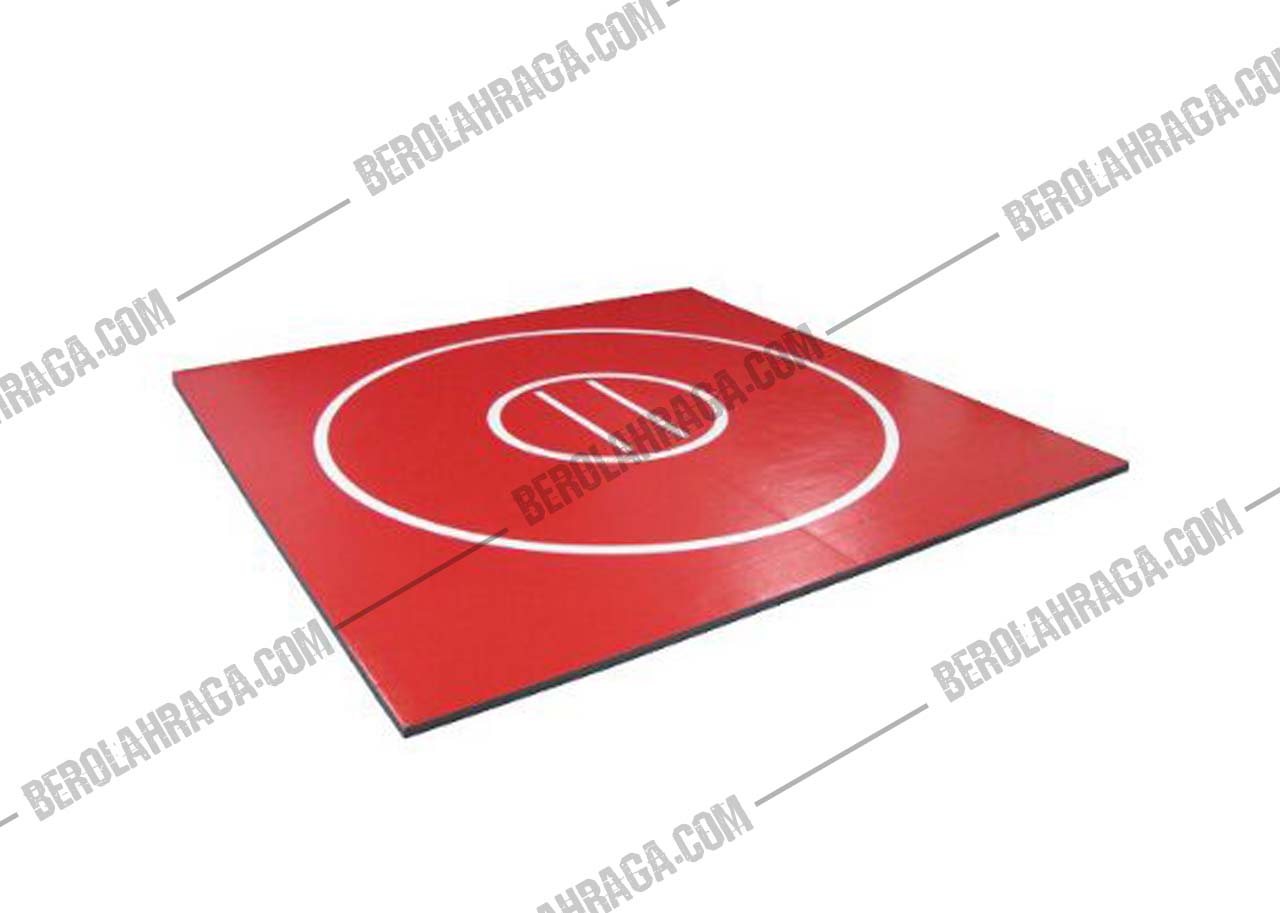The image depicts a large, flat, red square mat, likely used for sumo or wrestling purposes. The mat features black padding along the bottom edge. In the center of the mat, there is a distinct design consisting of two concentric white circles, with a smaller circle inside the larger one. Within the innermost circle, there are two parallel vertical lines. The surface of the mat appears slightly shiny, indicating a reflective material. Repeating across the entire image is a watermark that reads "berolahraga.com."